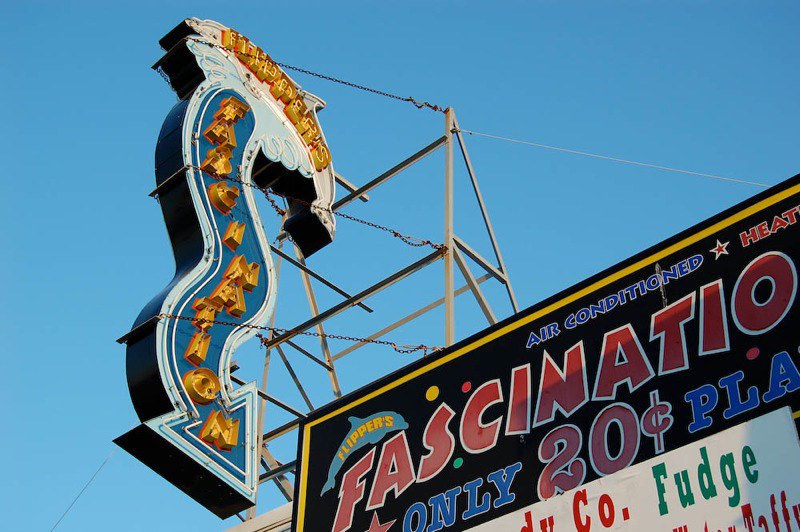This photograph captures the vibrant essence of a vintage carnival ride or arcade attraction. The image is dominated by a clear blue sky, enhancing the visibility of the multicolored signage displayed. Central to the scene is a sign with bright, bold colors, featuring yellow text on a backdrop of black, red, blue, and white hues. The fragmented text includes "air-conditioned" in blue, "flippers" in yellow on a blue dolphin, and "fascination" in red with a white outline. A distinctive feature is a blue, squiggly arrow outlined in white and pointing downwards, apparently reading "fascination" or a similar word. The sign declares "only 20 cents" in red text and hints at additional words like "fudge" and possibly "taffy". The signage is embellished with decorative elements including red stars and colorful dots. The metal frame and silver chains securing the sign are also visible, suggesting the sturdy structure's attachment to a roof or framework. This scene, with its potential for neon illumination and retro charm, encapsulates the allure and nostalgic appeal of mid-20th-century amusement park attractions.